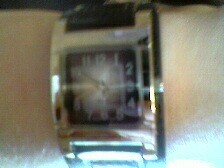This image features an up-close view of a wrist adorned with a wristwatch. The person's wrist, extending from the left edge of the frame to the right, displays very light or white skin. The wristwatch, which serves as the focal point, is distinctly square-shaped with a chunky, chrome silver-tone metallic finish that is both reflective and shiny. Despite the blurriness and light glare affecting the image, some details remain visible: the watch face is black with a gradient effect, fading towards the edges. Silver-tone numbers 1 through 12 encircle the black center, accompanied by silver-tone hands. 

The watch band appears to be dark, with varying descriptions suggesting it could be dark navy blue, black, or possibly dark brown. The image shows a small, thin black border at the top and a blue shine of light at the bottom, highlighting the band, which goes around the wrist. Additionally, a darker central border and a smaller inner square also seem to be present, though their exact colors are uncertain due to the image’s quality. The watch hands are difficult to discern precisely but seem to be positioned around the 10 and between the 8 and 9 marks. The photograph's blurriness and light glare make these details somewhat indistinct, yet the overall impression is of a stylish, metallic, square watch centered on a light-skinned wrist.